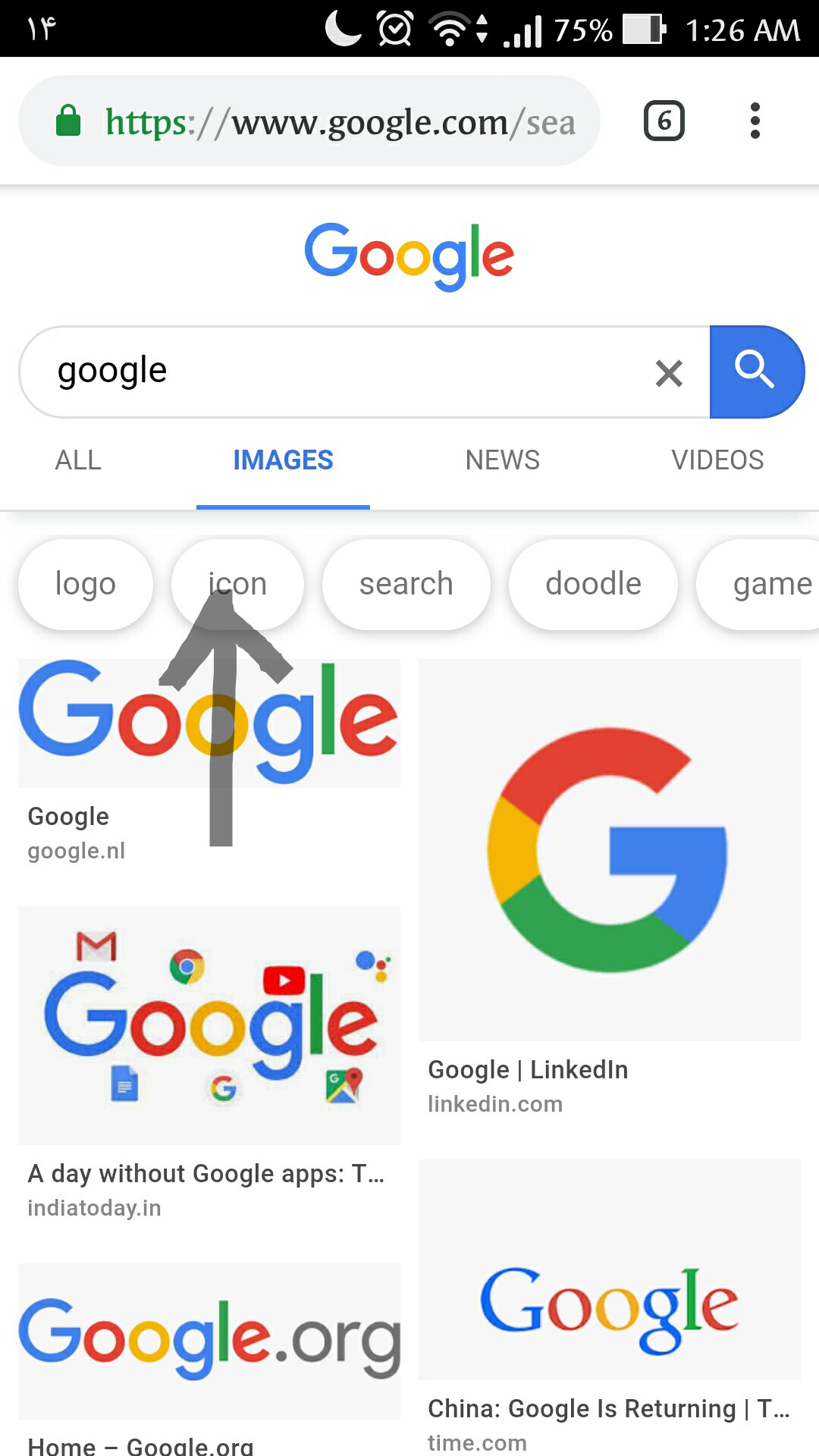The image is a screenshot featuring a predominantly white background. A black horizontal banner spans across the top, displaying various white icons including the time, battery level, reception signal, Wi-Fi status, and an alarm clock. Below this banner, a gray oval is seen with a green lock icon on the left, adjacent to green text "HTTPS" which transitions to gray text "://www.google.com/SEA". To its right, there is a dark black outlined square containing the number six, followed by an ellipsis (three vertically aligned dots).

A light gray horizontal line separates this section from the center-aligned Google logo that is rendered in its iconic multicolored letters. Beneath the logo, there is an oval-shaped search bar outlined in light gray with the word "Google" in black on the left and icons for a magnifying glass and an "X" on the right side. Below the search bar, a menu with options—All, Images, News, Videos—is presented. All options are in gray except for "Images," which is highlighted in blue and underlined.

Further down, there are several gray oval buttons labeled Logo, Icon, Search, Doodle, and Game. A hand-drawn black arrow points from below towards the "Icon" button. The remainder of the screen consists of various squares and rectangles, each containing either the word "Google" in the company's colors, "google.org," or a large "G" in the Google stylization.